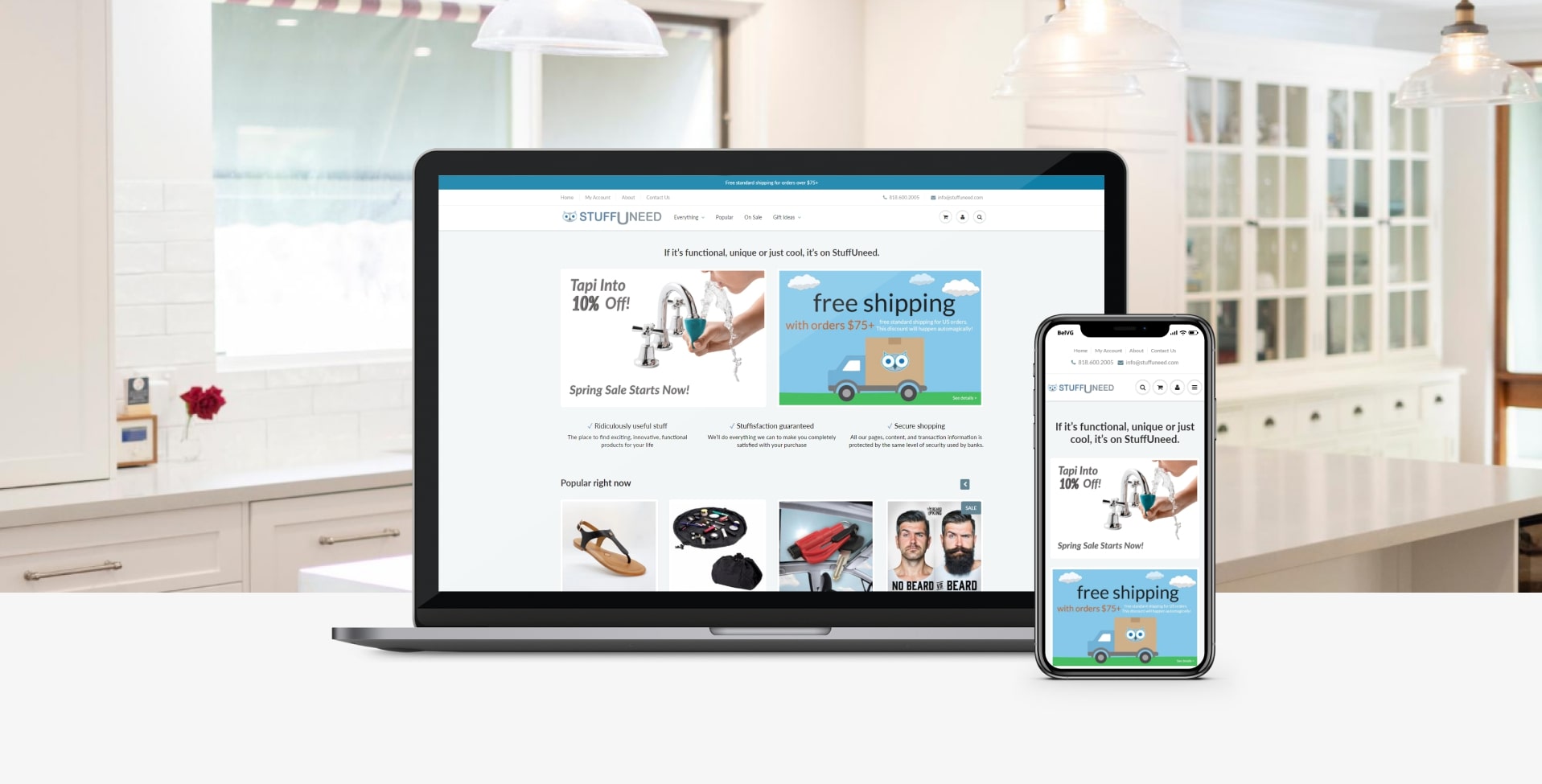This image appears to be part of an advertisement, perhaps a banner or a screenshot from an online ad. Dominating the scene is a laptop and a smartphone placed on a kitchen counter, promoting a website called "Stuff You Need." The website seems reminiscent of Chinese e-commerce platforms like Tennew and Wish.

The advertisement is predominantly white, featuring several snippets of information. Notably, it boasts "Free shipping with orders over $75." Surrounding the devices, the ad showcases a variety of products including:
- A fountain attachment that can be added to a faucet for drinking purposes
- A single shoe
- A work bag
- A bearded man, possibly modeling a product

The background depicts a pristine, white-themed kitchen, embodying a stereotypical country style often seen in affluent homes. The setting is stark and sterile, save for a single red rose in a jar by the sink, providing the only pop of color. The decor evokes a sense of wealth but lacks warmth and personality.

The smartphone's screen mirrors the content displayed on the laptop, highlighting the same "Stuff You Need" branding, the faucet attachment, an image of a woman drinking from it, and the free shipping message.

Overall, the ad exudes an aura similar to budget-friendly Chinese knockoff sites, raising questions about the origins and quality of the advertised products.